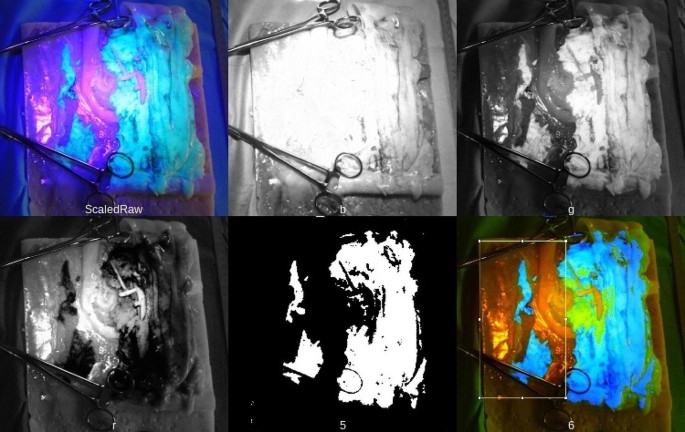The image depicts a series of six square-shaped renderings of a surgical tray, organized in a 2x3 grid format. Each rendering portrays two hemostats and an indeterminate mass of organic material positioned on the tray, akin to an Andy Warhol-style array where the same image is repeated with distinctive color filters. 

In the top left, the image is bathed in saturated blues and purples, labeled with the text "scaled raw." Moving to the top center, the rendering shifts to a blown-out black and white with high brightness, marked with a white letter "B." The top right image continues with a black and white theme but is considerably darker, showcasing more of the tray's contents and featuring the letter "G."

On the bottom row, the leftmost image presents a lower-contrast black and white view with less saturation, tagged with the letter "R." The middle bottom panel escalates the contrast significantly, rendering the image almost pitch black with striking white accents, labeled with the number "5." Finally, the bottom right image adopts a turquoise and brown filter with a detailed rectangle drawn around part of the content on the tray, annotated with the number "6."

This composition gives an impression of a disturbing and artistic representation of a medical scene, enhanced by varying visual manipulations that obscure the clarity of the organic material depicted.